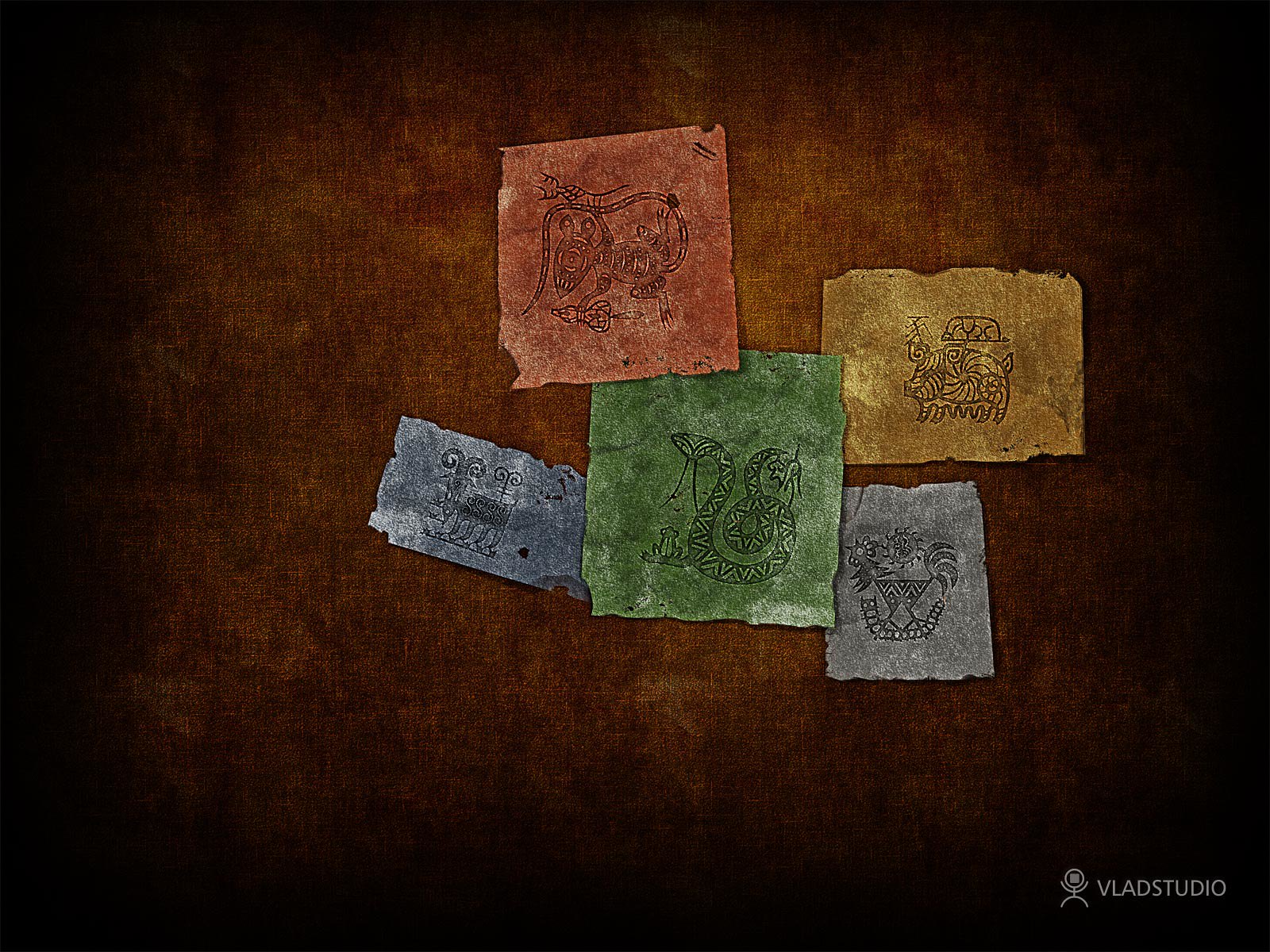This image presents a top-down view of a tabletop, possibly made of wood, with a central light source that illuminates the middle and leaves the corners dark. On this table, five distinctly colored and frayed pieces of material, either paper or cloth, are laid out. Each piece features simple, black ink drawings of animals, and they vary in color and size.

Starting from the top left, a blueish-purple piece displays a ram-like figure. Above this, a squarish brown piece depicts a rat holding a bottle, with its tail coiled elegantly. The largest piece, a green square in the center, shows a stylized snake coiled in geometric patterns. To the right, an orange piece features a lizard or crocodile drawing. Below, a grey piece presents the simplistic image of a rooster or chicken. Lastly, a yellow piece on the bottom right illustrates a pig, with the figure bearing spiral repeating lines.

These pieces rest on a dark brown backdrop, which might be a woven material or a wooden surface with a vignetted effect. In the bottom right corner of the image, a logo of a stick man with uppercase letters reading "Vlad Studio" is visible.